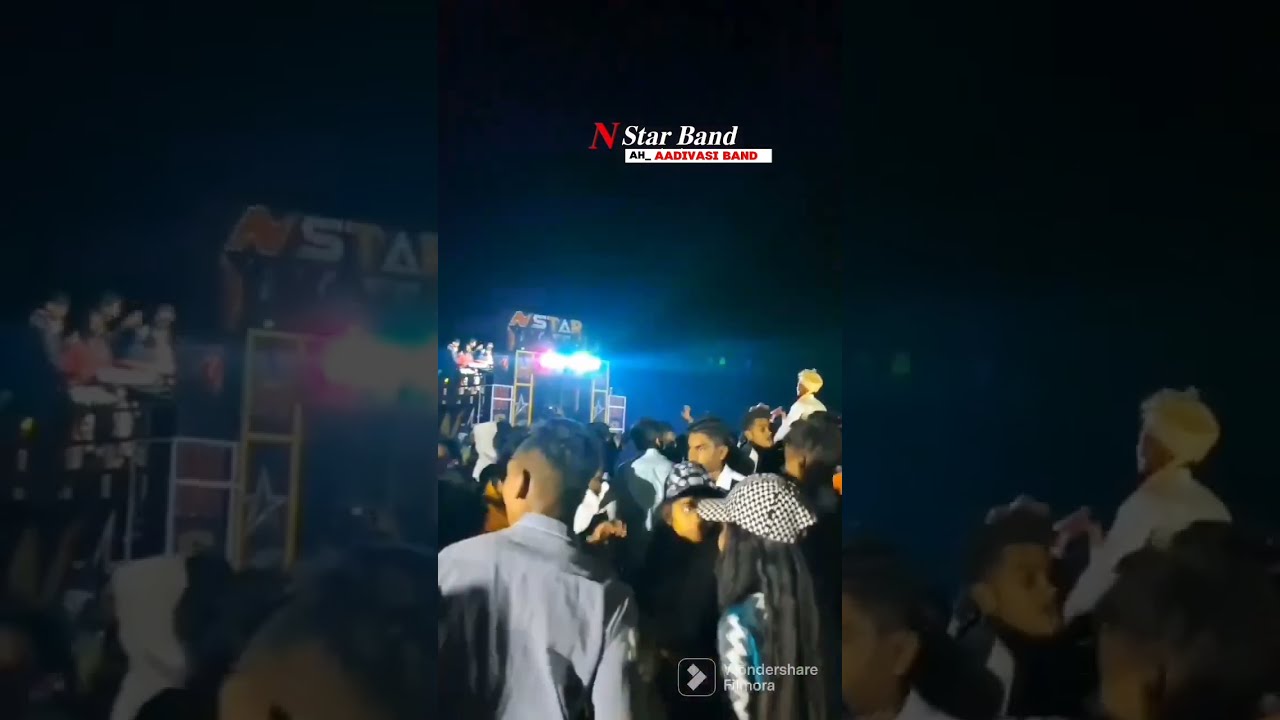In this detailed photograph of a concert, the image is divided into three segments with the central segment, shaped like a smartphone, serving as the focal point. The scene captures a vibrant mix of concert-goers, silhouetted against the dark backdrop illuminated by stage lights. To the left, a fence separates a sea of people, who are intently gazing to the right side of the image, where a colorful board prominently displays the word "STAR." The board emits blue and red lights, enhancing the festive atmosphere. Near the bottom left corner, a man in a long-sleeve blue polo shirt stands out, while on the far right, another individual in a bright yellow cap adds a dash of color. Amidst the crowd, one can spot a girl with long hair wearing a spotted baseball cap.

Above the crowd, on a banner, are the words "N Star Band" and a smaller line of text that reads "A-M-A-A-D-I-V-A-S-E, Atavace Band." The right and left segments of the image are slightly faded, giving focus to the vibrant middle where young people are milling around and chatting, some dancing and others simply enjoying the ambiance. The entire scene is bathed in an eclectic mix of colors from the stage lights, adding to the lively and energetic vibe of the concert.